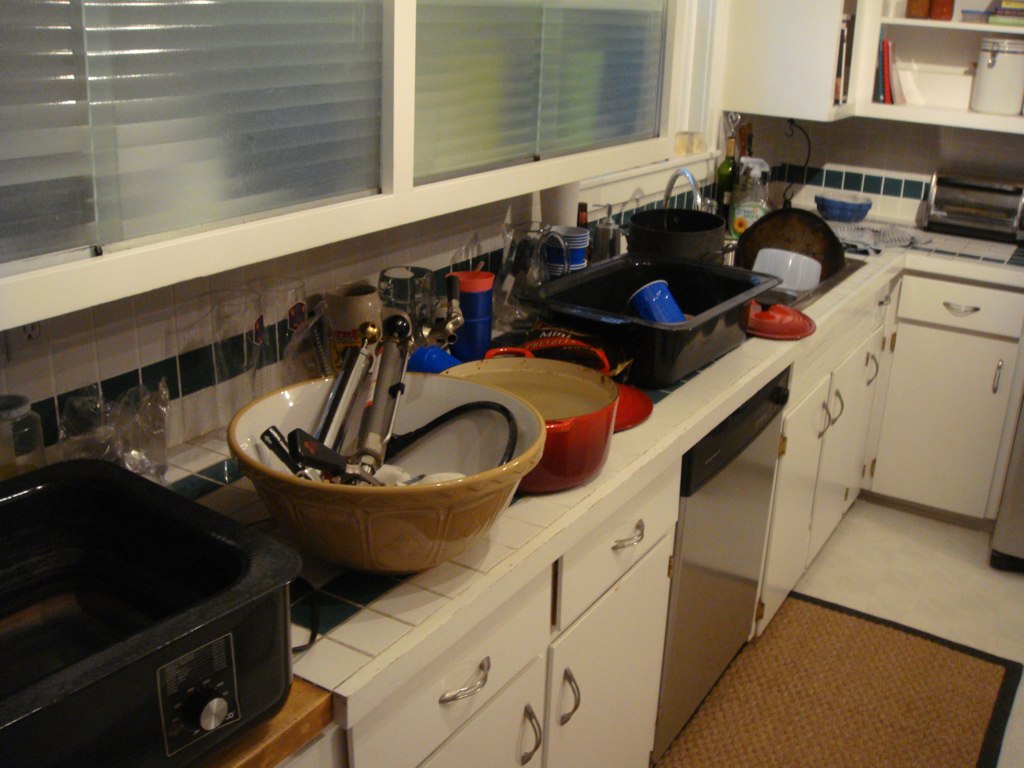In this photograph, we see a cluttered kitchen counter teeming with a variety of everyday items. The counter itself has a distinctive pattern in shades of white and forest green. A tan ceramic bowl occupies a prominent position, next to a well-used red pot that has visible stains. Scattered around are several glasses, blue solo cups nested in a roaster pan, and a green wine bottle. The silver sink faucet stands out, accompanied by a mix of black and pale gray dishes within the sink. A clear spray bottle with a flowered label sits nearby.

The countertop also features a blue ceramic bowl and a silver toaster oven. Overhead, the white cabinets, which are adorned with silver hardware, have open doors, revealing various stored objects inside. The floor below is white, and a tan mat with a black trim is centered in front of the sleek silver and black dishwasher adjacent to the sink, completing this detailed snapshot of a bustling kitchen space.